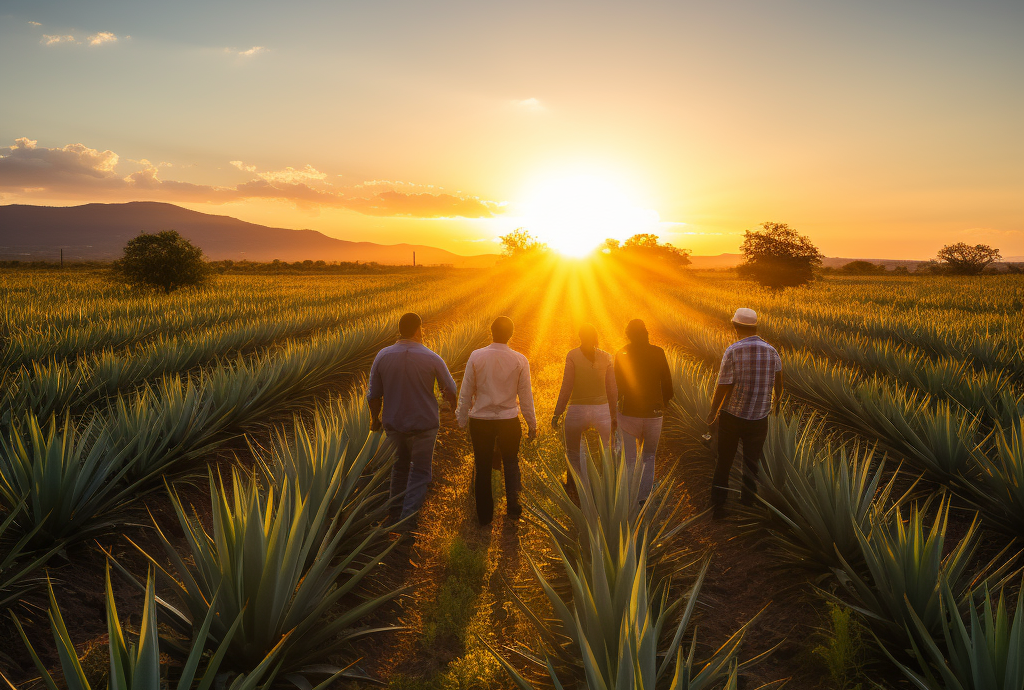In this rectangular, highly detailed photograph, five people stand in a row, their backs facing the camera. They appear to be in a desert-like farmland, surrounded by rows of agave plants, which have large, green, triangular, spiky leaves. The scene is set against a breathtaking sunset, with the sun sitting over the horizon at the center of the photo. The sky is ablaze with bright orange and yellow hues, accented by some scattered clouds. To the left, a small mountain range rises in the distance, while smaller hills and perhaps towers or windmills can be seen on the right. The landscape is dotted with occasional small trees and possibly power lines. The individuals are dressed in long pants; four of them wear long-sleeved shirts, while the fifth person, standing on the right, sports a short-sleeve plaid shirt and a hat. They seem to be either walking through or standing among the rows of agave plants, mesmerized by the stunning sunset unfolding before them.